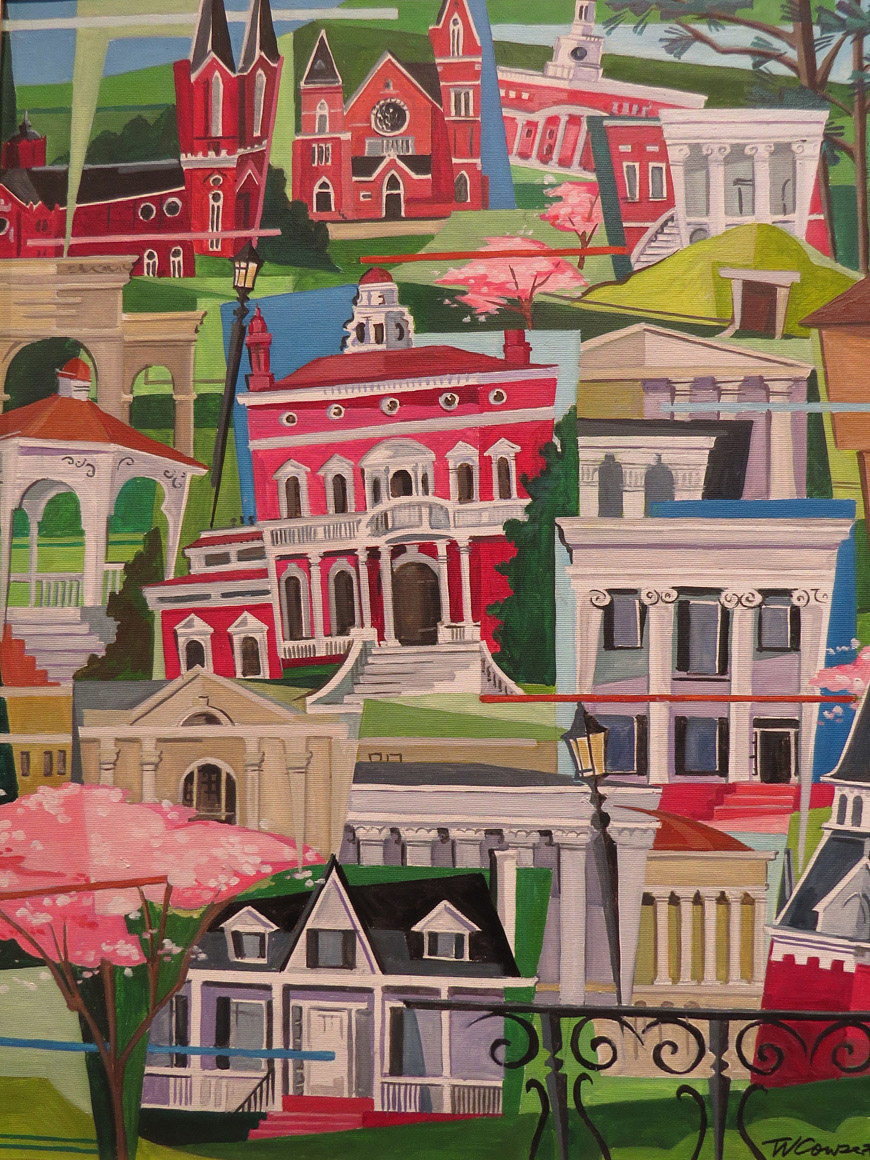The image is a photograph of a detailed painting depicting a vibrant collage of various buildings arranged closely together. The style appears to blend elements of both traditional and cartoonish art, creating a unique and colorful townscape. The buildings are predominantly Western in architecture, featuring diverse facades that include porches, columns, and colorful exteriors in shades of white, red, blue, tan, and brown.

In the foreground is a notable two-story house with a front porch, surrounded by white railings and red steps leading up to a white door. The house is primarily blue with a dark blue sloped roof. Scattered throughout the painting, recognizable landmarks such as schools, churches, and residential houses create a sense of familiarity and nostalgia.

Adding to the picturesque scenery, pink Sakura trees with white flowers are strategically placed, suggesting a serene, yet somewhat surreal setting. Lamp posts are interspersed amongst the buildings, adding a delicate touch of everyday life. The painter's signature, T.W., is subtly inscribed in the bottom right corner, while the overall composition gives the impression of a cohesive yet fantastically eclectic town portrait.